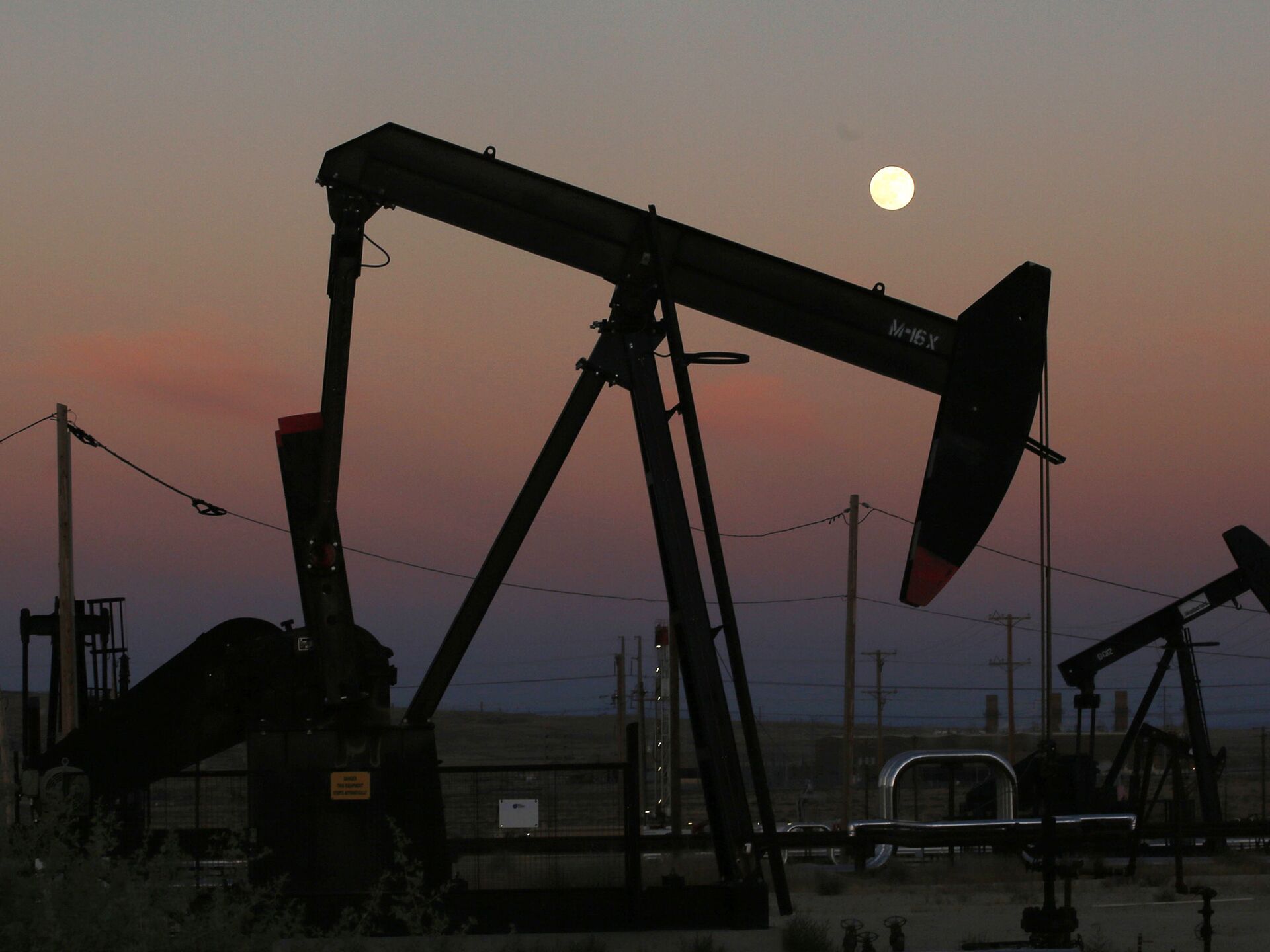This image is a color photograph with a landscape orientation, capturing a construction site in a style of photographic realism. The focus of the image is an oil well pump, centrally positioned atop a metal tripod support that resembles an upside-down V. The pump has a bent arm: the right part of the arm rests on the tripod, while its head rotates and drills into the ground, appearing as a massive hammer-like device.

In the background, several power lines and poles are visible, stretching across the horizon. There are additional oil drilling pumps silhouetted against the sky, backlit by the setting sun. The sky itself transitions in an ombre gradient from gray at the top to bands of orange, pink, and blue near the horizon. A perfectly white moon is situated near the top right of the image, adding a serene touch to the otherwise industrial scene. The bottom 20% of the photograph is land, depicted in dark tones due to the low light, with parts of the oil pump partially cropped at the bottom left.